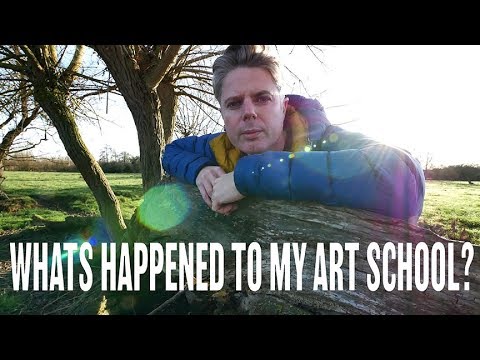The photograph features a middle-aged man wearing a blue winter coat with a mustard-yellow lining, leaning over a large, fallen tree trunk with his elbows resting on the log and his arms spread outward. He has a puzzled expression as he gazes directly at the camera. The image is framed by thick black letterbox bars at the top and bottom. The background reveals an overcast sky, a grassy field, and two barren trees to the left, with more leafless trees visible at the far edge of the scene. Bold white capital letters at the bottom of the image caption it with the question, "WHAT'S HAPPENED TO MY ART SCHOOL?"